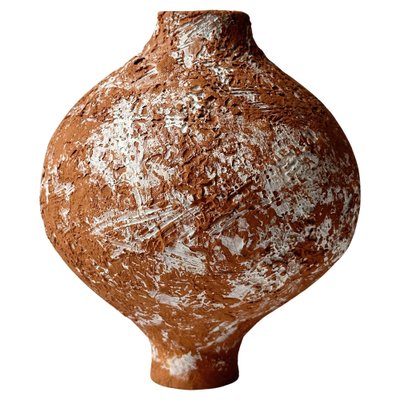This color photograph vividly showcases an ancient pottery artifact set against a brightly lit, plain white background, reminiscent of images found in museum catalogs or displays. The vessel appears to be meticulously crafted from terracotta clay, exhibiting an earthy orange hue intermixed with patches of white, possibly remnants of its original coating that have worn away over time. The base of the artifact is notably small, presenting a potentially top-heavy form which stabilizes the vessel with a narrow foot. As it ascends, the body of the pot swells into a nearly spherical, bulbous shape, adorned with sgraffito scratch marks and a couple of bands of design around its shoulder. This rough-textured vessel tapers into a narrow neck, slightly wider than its base, featuring the same earthen tones and rough design that give it a distinctive ancient feel. Despite its crude and uneven construction, this artifact's form and texture suggest it might have been used to hold water, combining practical utility with artistic craftsmanship.